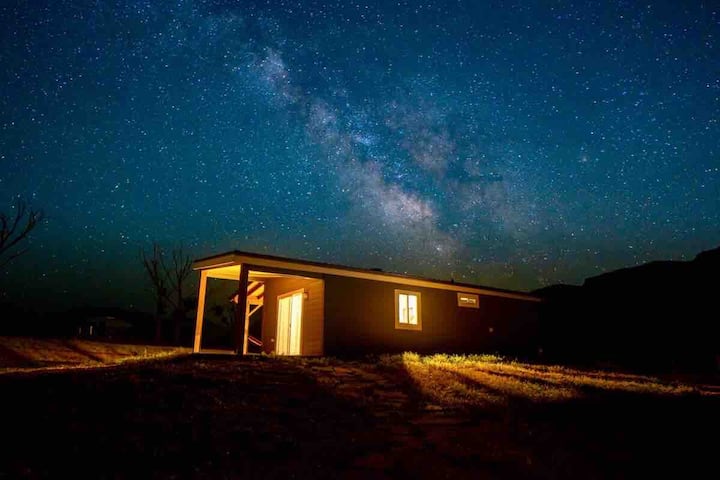A captivating nighttime photograph showcases a small, likely residential building bathed in warm, inviting light that spills out onto the porch. The house itself is painted a barn red with contrasting white trim along the edges of its black roof. Set against a stunning backdrop, the Milky Way stretches across the sky in mesmerizing shades of dark to light blue, indicating that the photo was taken shortly after sundown. The stars are abundantly scattered across the sky, revealing a pristine night untainted by light pollution. The surrounding landscape features barren trees with scant leaves, suggesting a time of year that could be early spring or late fall. Sparse patches of grass encircle the house, hinting at an arid, rural, or even desert-like location, far removed from the hustle and bustle of urban life.